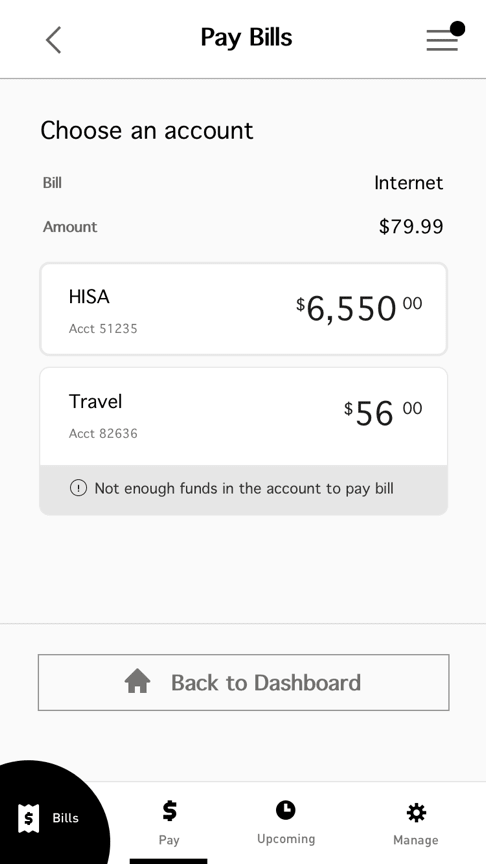The screenshot captures a "Pay Bills" interface from a financial management application. At the top, it prompts the user to "Choose an Account." On the right, a list of bills is displayed, starting with "Internet" at an amount of $79.99. Below, it lists several accounts:

- **HISA Account (51235):** Balance of $65.50
- **Travel Account (23826):** Balance of $56.00 with a notation: "Not enough funds in this account to pay bill."

At the bottom, there are several options, including "Back to Dashboard" and buttons for "Dollars," "Bills," and "Upcoming" under a section labeled "Retail Pay." A "Manage" button is also visible. The overall impression conveys a system designed for tracking and paying bills, highlighting account balances and payment capabilities.